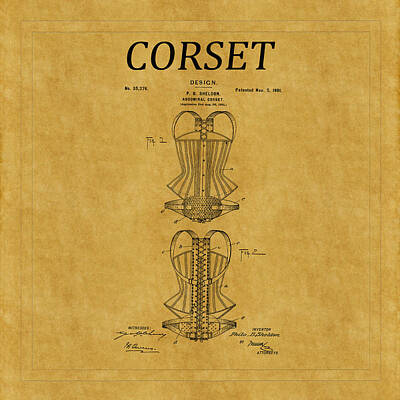This image displays a vintage yellowed piece of paper, possibly aged or stained, featuring a detailed patent for a corset. At the top of the page, the word "CORSET" is prominently displayed in large, black, all-capital letters. Just below "CORSET," the word "Design" appears in smaller print. To the left of "Corset" is a number that appears to be 35,378 or 35,376, and to the right of "Design" is a partially legible publication date. The center of the page is dominated by two detailed black outlines: one illustrating the front view of the corset, and the other, positioned below, showing the back view, where the corset ties. Scattered across the corset are various numbers and letters marking different points and components. At the bottom of the page, to the left and right of the back view image, are four signatures—the inventors or patentees. The entire document appears to be hand-signed, enhancing its historical and authentic appearance.